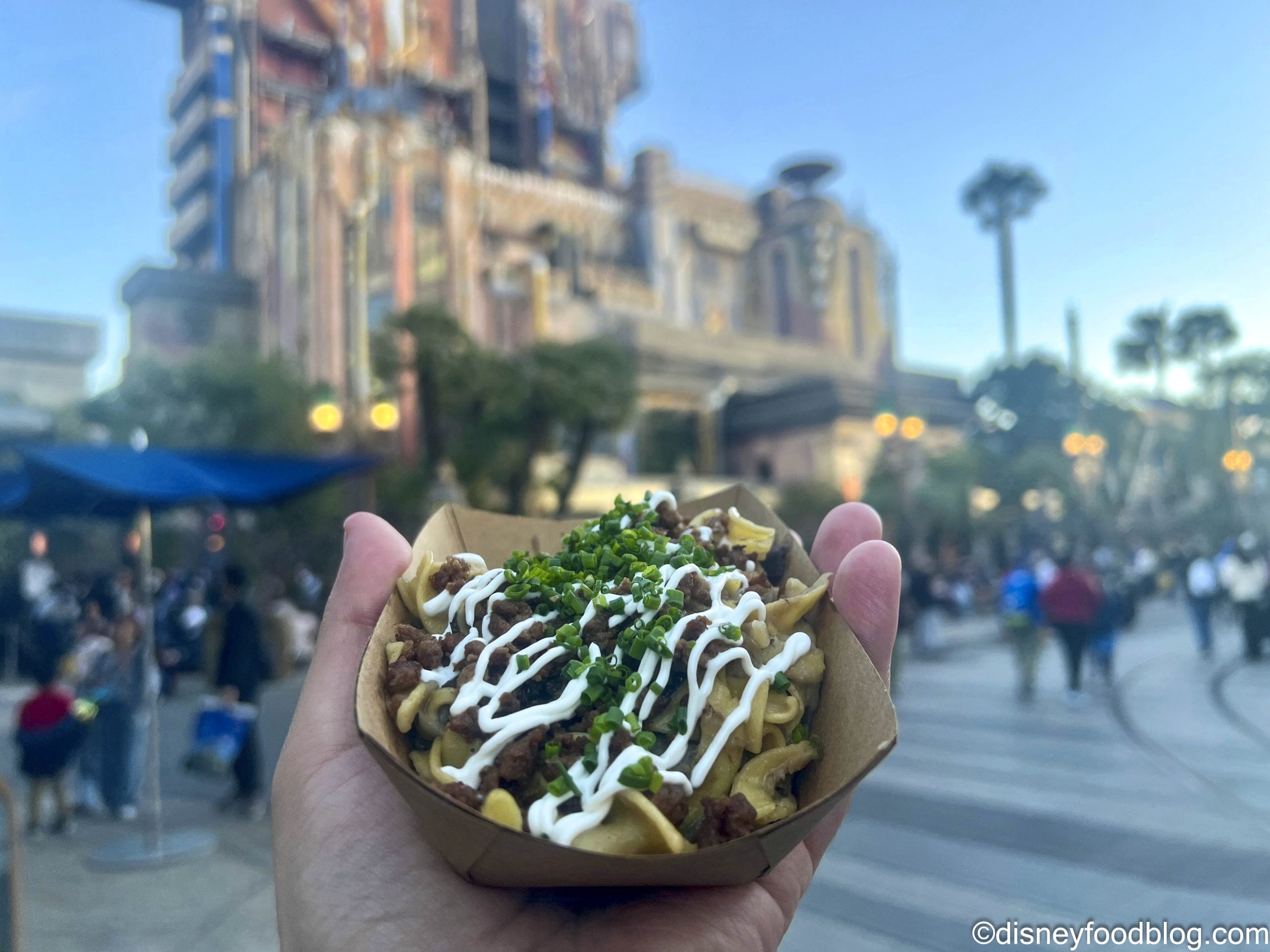In the foreground of this vibrant outdoor photograph, a man is holding a brown paper bowl filled with a mouthwatering dish that combines crispy chips or pasta with savory chopped meat, all generously drizzled with a white sauce and garnished with thinly sliced green onions or chives. The bottom right corner of the image is marked with a watermark reading DisneyFoodBlog.com, adding a professional touch. 

The background hints at the bustling atmosphere of Disneyland, with a walkway crowded with visitors and various buildings, including a towering structure reminiscent of the Hollywood Tower, known for its thrilling rides. Further adding to the scenic charm are palm trees on the right and a castle-like building in the distance, all under a bright, cloudless sky. Although slightly blurred, the backdrop captures the essence of a lively Disney park setting during a sunny day, complete with features like blue shade coverings and tall tram supports visible amidst the crowd.